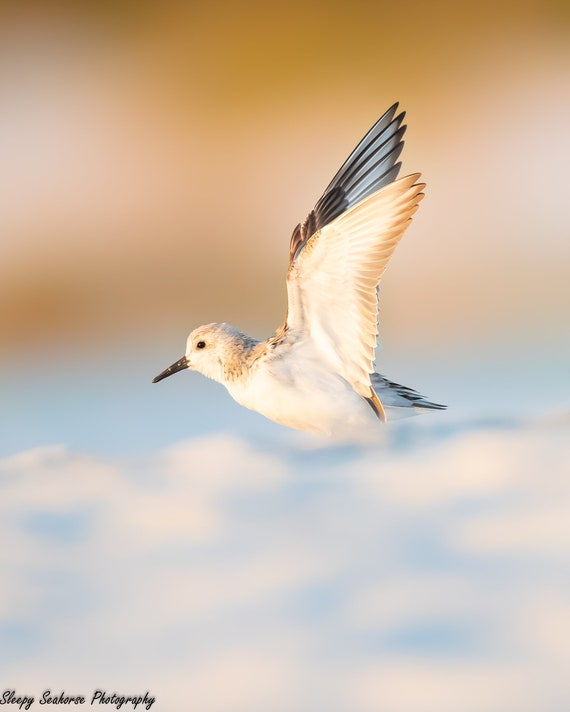This is a stunning photograph of a white bird in flight, captured in sharp detail against a dynamic and colorful sky. The bird is in profile, presenting its left side prominently with a dark beak and a dark eye. Sunlight reflects off its form, highlighting the underside of its opposite wing, which displays shades of gray interspersed with some brown at the tips. The bird's wings are angled upward, showcasing large white feathers transitioning to darker hues toward the edges. The sky behind the bird is a beautiful gradient of light blue and white puffy clouds, transitioning to tones of orange and bronze, suggesting a sunset occurring above the clouds. The bird is centrally positioned, and the overall scene is enriched with an out-of-focus backdrop blending blue sky and clouds at the bottom, with a brown and pink undertone at the top. In the bottom left corner, the words "Sleepy Seahorse Photography" are elegantly inscribed in black script, adding a signature touch to the photograph.